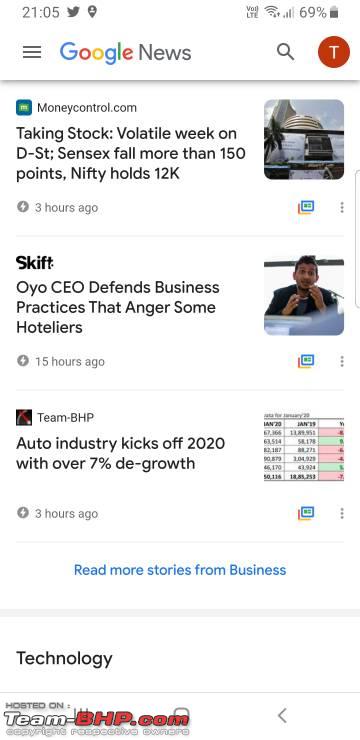This screenshot captures a Google News feed displayed on a mobile device. The device's status bar at the top reveals it is 9:30 AM and shows several indicators: a Twitter notification icon to the right of the time, followed by the Voice over LTE (VoLTE) icon, Wi-Fi signal strength, network signal bars, and the battery percentage at 69%.

The news feed begins with a headline from Moneycontrol.com, detailing a turbulent week in the stock market with the Sensex dropping by over 150 points and the Nifty index reaching 12,000. This article was published three hours ago. The next headline is from Skift, featuring OYO's CEO defending the company's controversial business practices, an article posted 15 hours ago. Following this is a news piece from Team-BHP discussing the auto industry's strong start to 2020, boasting a growth of over 7%, also posted three hours ago. The page invites users to read more business stories and notes that technology-related articles are sourced from Team-BHP, with all content under respective copyrights.